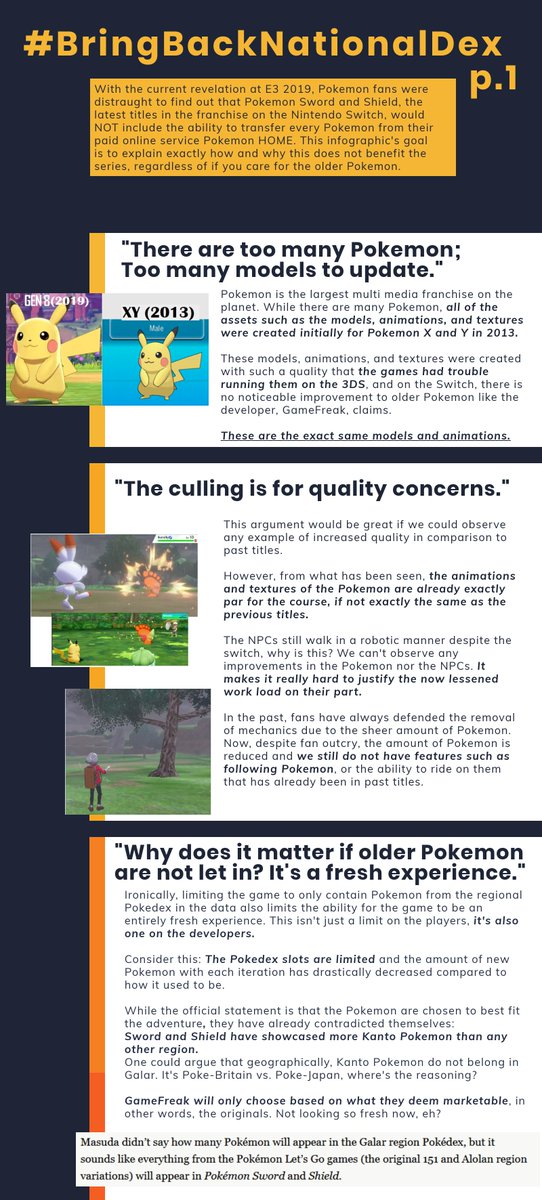"Bring back the natural Dex!" A passionate Pokémon fan voices their frustrations over the current direction of the franchise. The Pokémon series, the largest multimedia franchise on the planet, has amassed an enormous roster of creatures over the years. However, despite the vast number of Pokémon, the models, animations, and textures were initially created for Pokémon X and Y back in 2013. The recent "culling" of Pokémon from newer titles is claimed to be for quality reasons, but this argument holds little weight when examining the games.

The animations and textures of Pokémon have not shown significant improvement compared to older titles, with many appearing unchanged. NPCs still exhibit a robotic mannerism, even on the more powerful Nintendo Switch. This lack of observable improvements makes it challenging to justify the reduced workload on the developers' part. Previously, fans defended the removal of certain mechanics due to the sheer number of Pokémon, but now, despite the reduced roster, features like following Pokémon are still absent.

The exclusion of older Pokémon limits not just the player's experience but also the developers' creative potential. While the official statement claims Pokémon are chosen to best fit the adventure, contradictions are evident. For example, Pokémon Sword and Shield feature a disproportionate number of Kanto Pokémon, despite them being geographically misplaced in the Galar region, which is inspired by Britain, contrasting Kanto’s inspiration from Japan.

The outcry is about more than just nostalgia; it's about preserving the integrity and richness of the Pokémon journey. Such decisions, fans argue, stifle the series' potential and limit the freshness of new adventures. The Pokémon Company’s choices have left many fans yearning for the return of the complete National Dex and a truly expansive game experience.